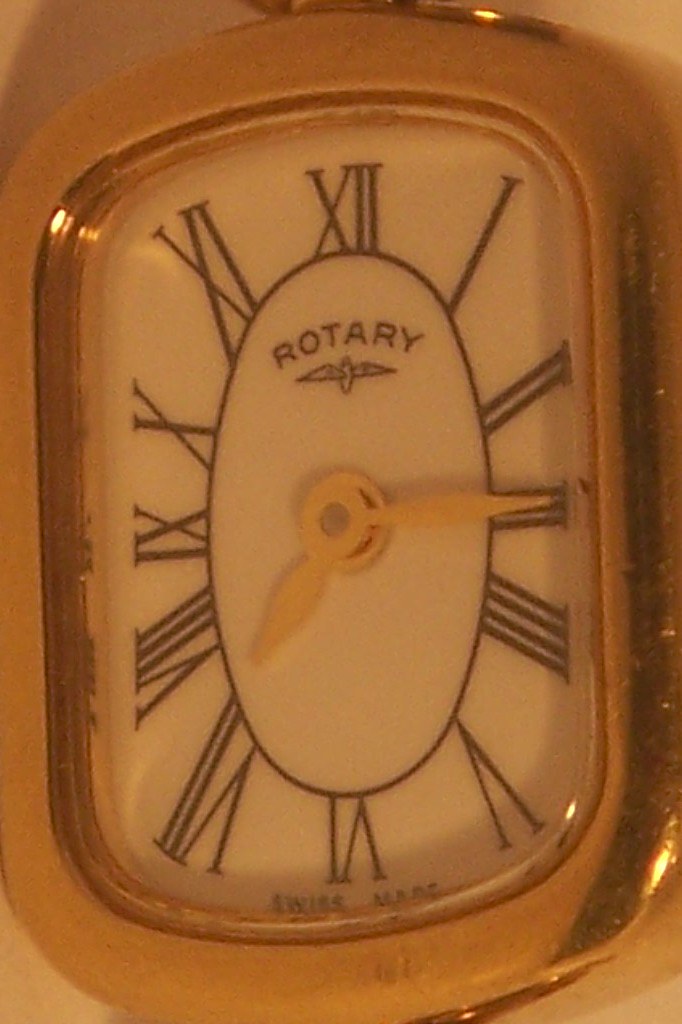This close-up image showcases a clock face dominated by a golden frame, prominently set against what appears to be a white wall. The golden frame, an elegant rounded rectangle approximately 1.5 to 2 inches thick, encapsulates the clock, adding a touch of opulence to its design. The clock face itself is adorned with Roman numerals, each elegantly perched atop a continuous black oval encircling the clock's center. Both the hour and minute hands, crafted in gold, align gracefully to display the time as approximately 7:15. A subtle yet distinctive detail is the black text "Rotary" positioned in the upper middle section of the clock face, adding a refined brand touch to this sophisticated timepiece.